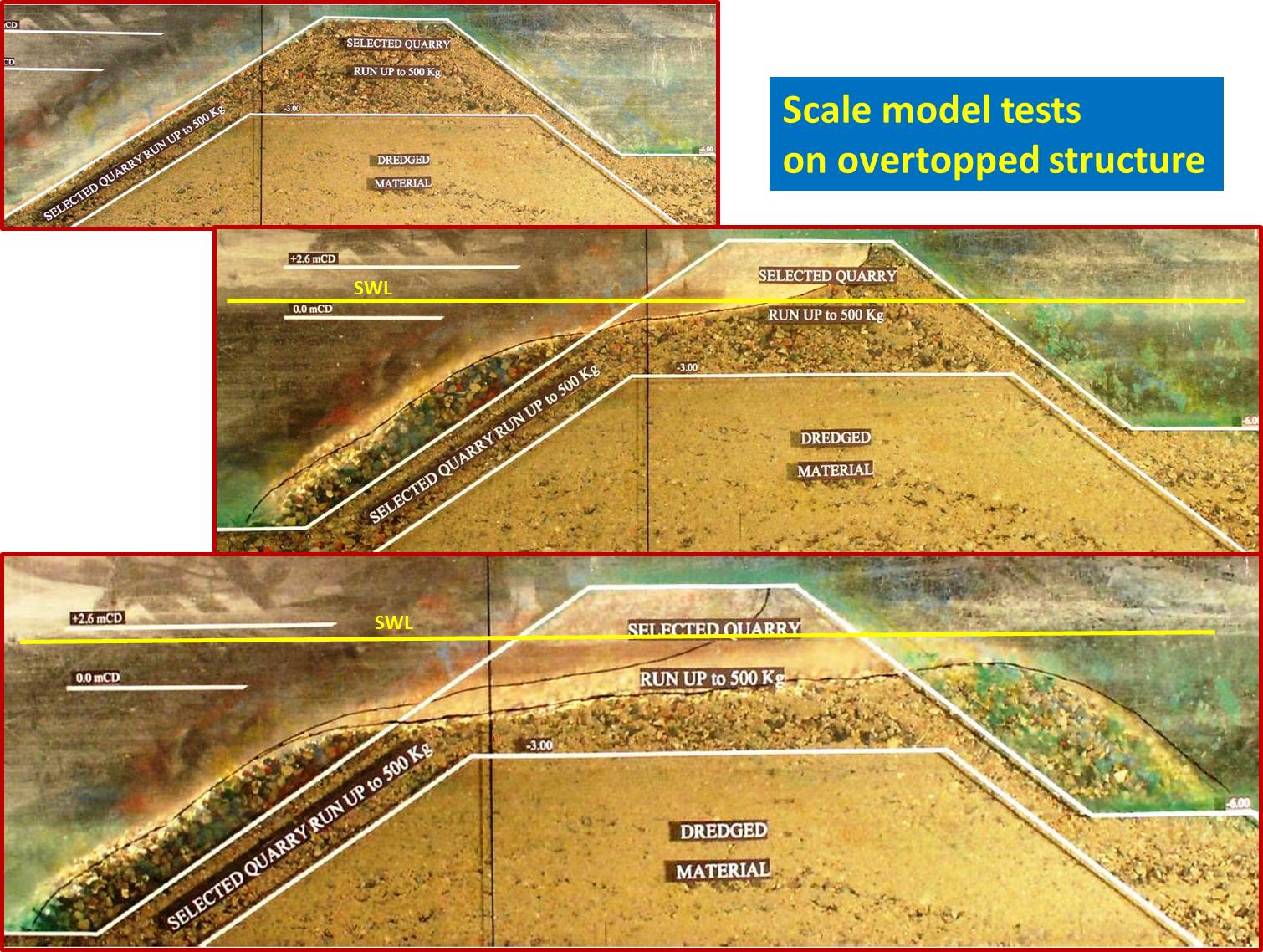The image features a detailed representation of an island's stratigraphy or sectional model with an emphasis on various layers of geological materials. In the top right corner, a blue rectangle contains the text "Scale Model Tests on Overtopped Structure," written in bright yellow. The layered composition of the island includes three sections: at the top, the label "Selected Quarry, run up to 500 KG" appears, repeated for emphasis; further down is another "Selected Quarry, run up to 500 KG"; and finally, at the bottom, "Dredged Material." Through the middle of the image, a prominent yellow line is present, labeled "SLWL." Accompanying this is a white line atop a brown box that states "+2.6 MCV," and beneath it, another white line indicating "0.0 MCV." The background features a mix of browns, greens, and blues, contributing to the island's textured appearance. Each stratified segment appears in a series of three consistent images, with the sections enlarging progressively from top to bottom.